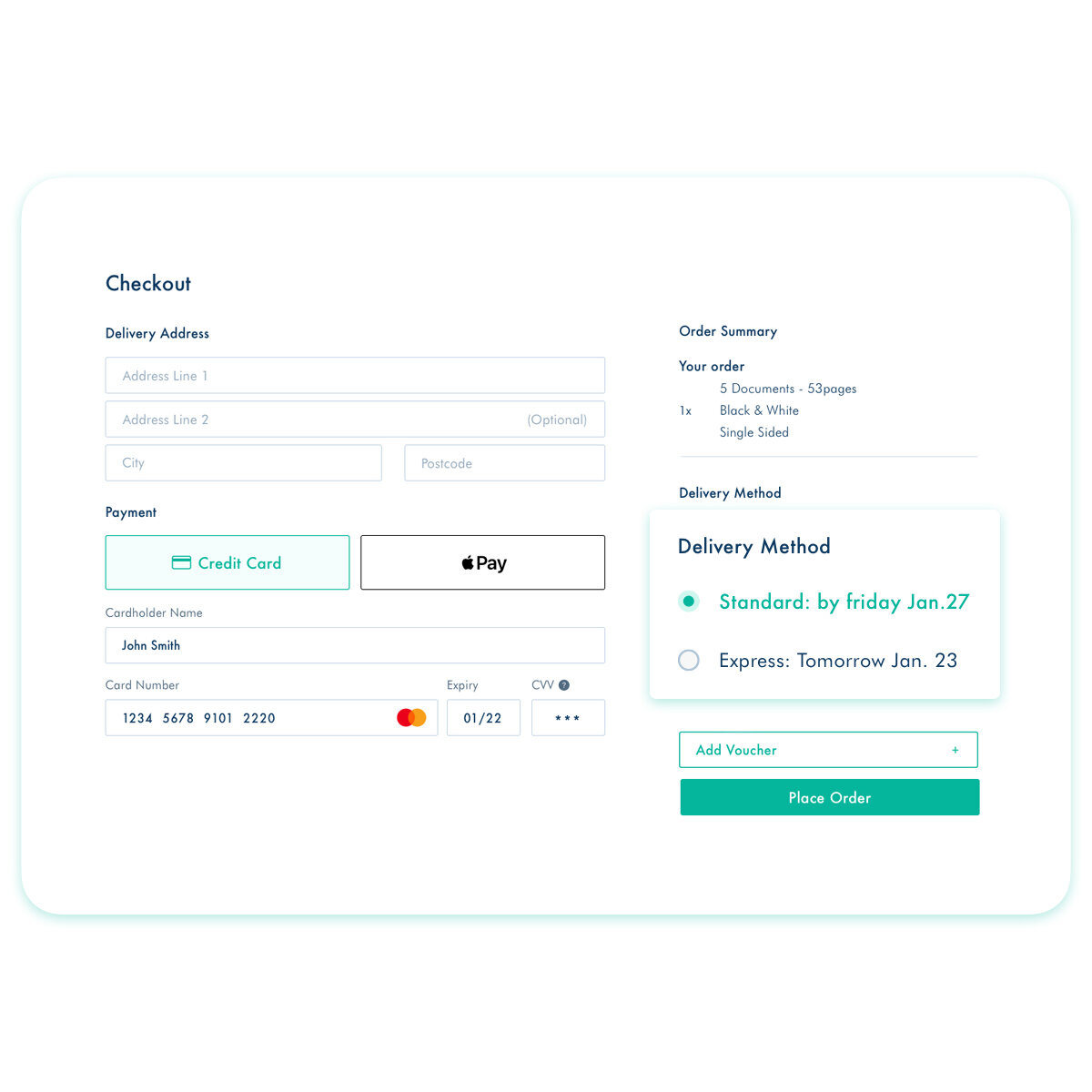The checkout webpage features a predominantly white background with black text and detailed sections for completing a purchase. The header reads "Delivery Address," with blank fields for 'Address Line 1,' 'Address Line 2,' 'City,' and 'Postcode Area.'

Below the address section, the "Payment" options are displayed. The "Credit Card" option is pre-selected and highlighted in green. Another available payment option is "Apple Pay," indicated by an Apple icon followed by the word "Pay." For the credit card details, the form includes fields for 'Cardholder Name' (pre-filled with 'John Smith'), 'Card Number' (displayed as '1234 5678 9101 2200'), 'Expiration Date' ('01/22'), and a CVV field with three dots, representing the security code input.

To the right, the "Order Summary" section lists the items, specifying "five documents, three pages each, black and white, single-sided." There are delivery method options: "Standard," arriving by Friday, July 27th, and "Express," arriving tomorrow, January 23rd. Below the delivery methods is an option to "Add a Voucher" highlighted in green text with a corresponding input box with a green outline.

The final step is the "Place Order" button, a teal green button with white lettering. Overall, the webpage design is clean and functional, intended for users to efficiently complete their document purchase.